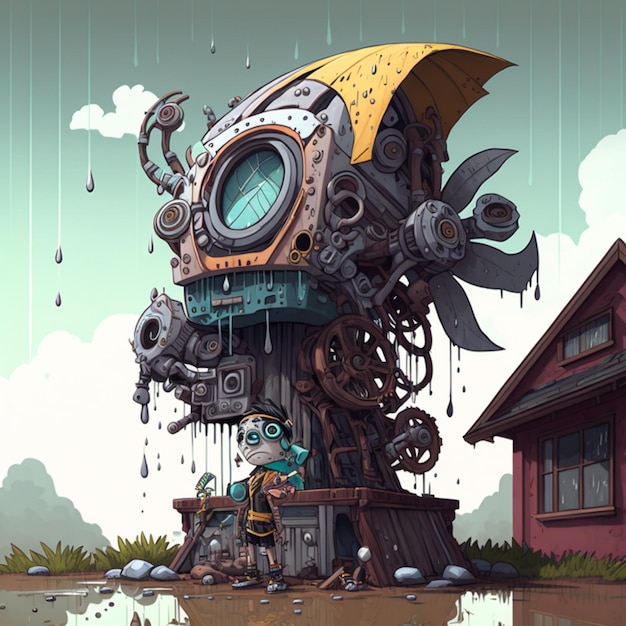The image depicts a cartoon or anime-style hand-drawn scene with a heavily detailed, futuristic machine as the central focus. The machine is blue and yellow, with various mechanical parts, including large cogs, wheels, and a giant fan or propeller on its right side. It also features a circular window at the top and seems to be a composite of wooden elements at its base, transitioning into metal, glass, and engine parts toward the upper section. The scene is set amidst a raining sky, with raindrops visibly falling onto the machine and forming puddles on the ground around it.

Standing in front of this impressive contraption, which could be some kind of advanced farming equipment or treehouse, is a boy with black hair, distinctive short legs, and a very sad expression on his face. He wears a black and orange outfit, perhaps indicating a connection to the machine, possibly as its owner or operator. The background includes large, bushy trees or a small mountain, enhancing the natural ambiance. 

Additionally, there are noticeable structures in the scene. On the right side of the image, a small, red house with windows on both floors stands near the contraption, while another description cites a purple A-frame house. The overall color palette and design elements create a dark, somber setting with overcast clouds contributing to the melancholic mood of the illustration.